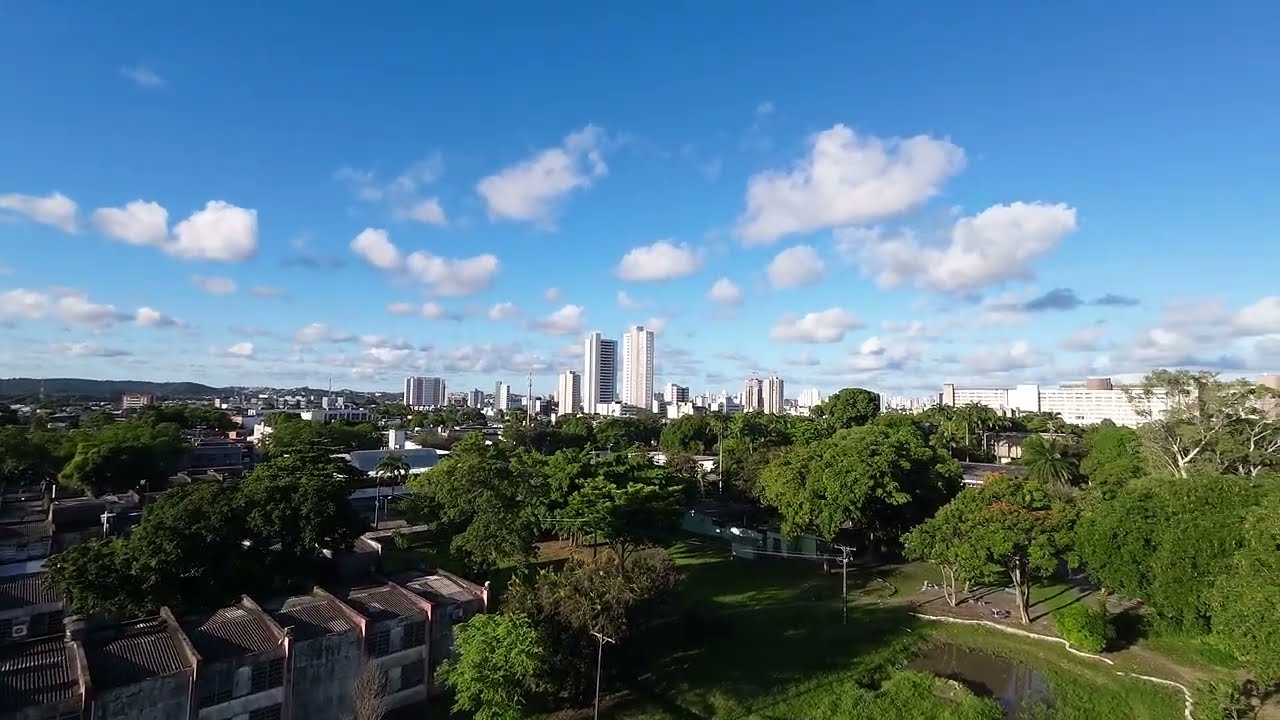The image depicts a horizontally aligned rectangular scene taken from an elevated perspective, showcasing a juxtaposition of urban and natural elements. The top half of the picture is dominated by a beautiful sky transitioning from bright blue at the top to a paler hue near the horizon, adorned with puffy white clouds that are densest near the horizon. On the horizon, a cityscape emerges with several tall, white and gray skyscrapers punctuating the skyline, flanked by shorter office and residential buildings.

In the foreground, particularly on the left side, there are older, somewhat run-down apartment buildings characterized by rusted, metal rooftops. The lower portion of the image is lush with greenery, featuring several average-sized, leafy green trees spread throughout. On the right side, a small, muddy pond sits in a grassy area with a white squiggly walking path beside it. The vibrant trees and foliage provide a stark contrast to the more subdued urban structures, creating a balanced and detailed portrayal of the blend between city life and nature.